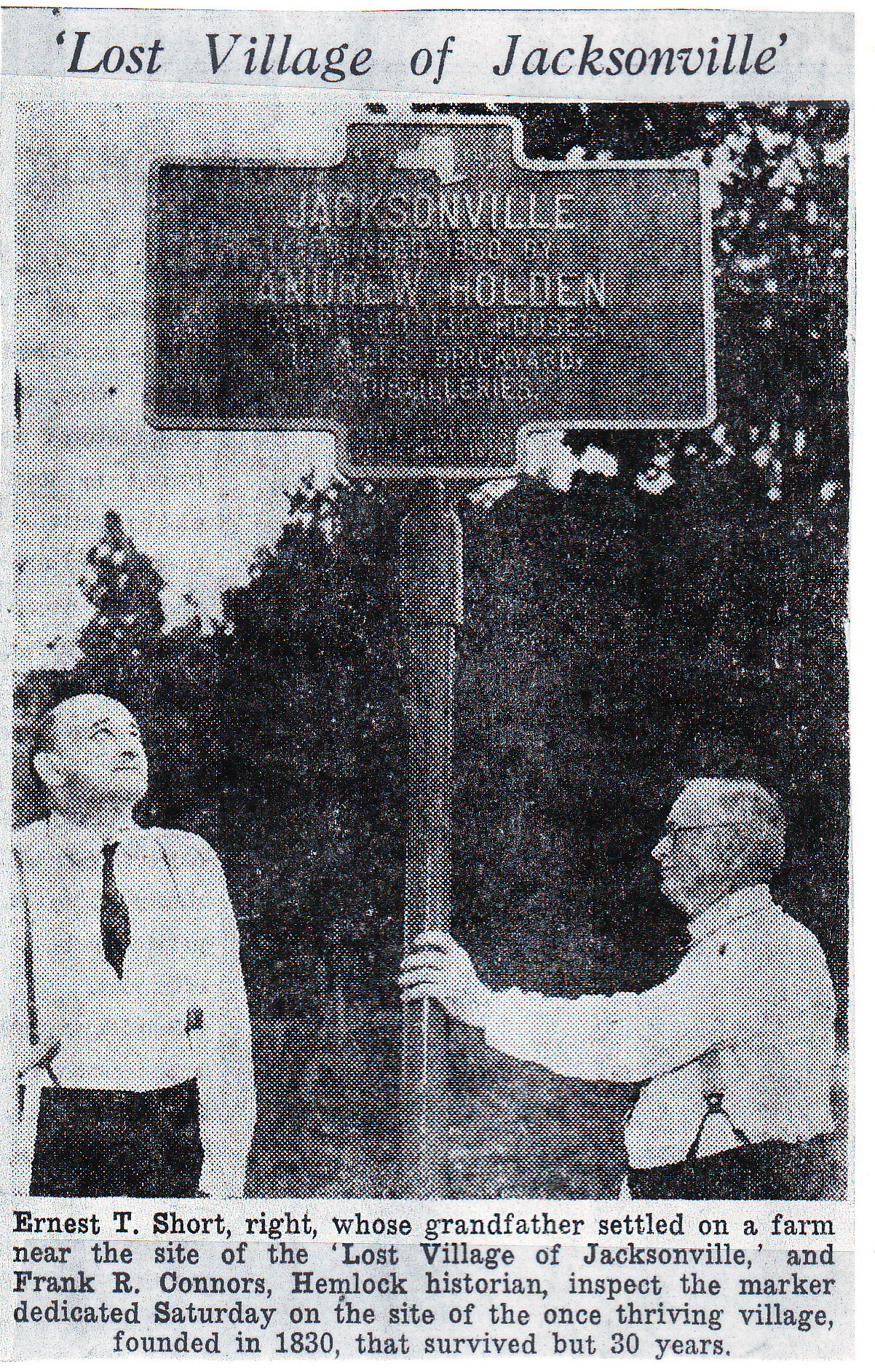This black-and-white newspaper photo, grainy and slightly blurred, captures a historic moment under the heading "Lost Village of Jacksonville." At the top of the image, a caption reads, quoted and prominently displayed. Two men stand beside a sign that marks the site of the once-thriving village, which was founded in 1830 by Andrew Holden but survived only 30 years. On the right, Ernest T. Shortwright, whose grandfather settled near the center of Las Vegas in Jacksonville, holds the sign with his left hand. He is dressed in a white shirt, black pants, and suspenders. On the left, Frank R. Conner, a historian from Hemlock, looks up at the marker. He is also wearing suspenders, paired with a black tie and white shirt. Behind them, faint outlines of trees merge with a cloudy sky, adding to the nostalgic aura of the photograph. The bottom caption informs readers that this marker was dedicated on a Saturday, highlighting the historical significance of a village long forgotten.